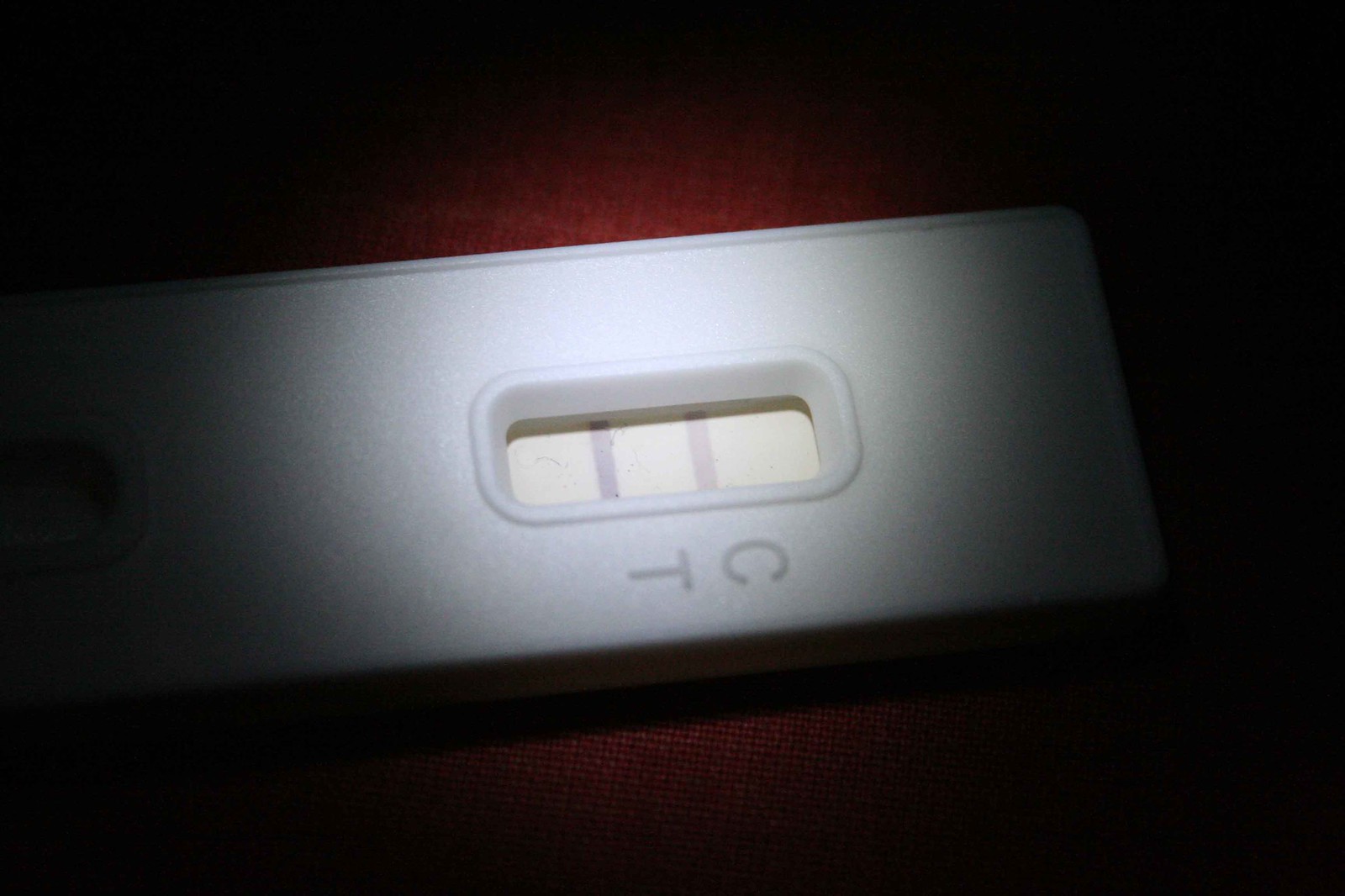A close-up image of the central portion of a COVID-19 test kit, illuminated under a spotlight. The test kit, pristine white, is placed against a vibrant red background, contrasting starkly with its surroundings. In the center, a rectangular viewing window prominently displays the test results, marked by distinct lines. The 'C' line, tinted with a pinkish hue, and the 'T' line, bearing a purplish color, are clearly visible. However, no legend or instructions are present to explain the significance of these lines. To the far left, the faint outline of an oval-shaped section of the kit adds a subtle hint of intricacy to the otherwise minimalistic design.